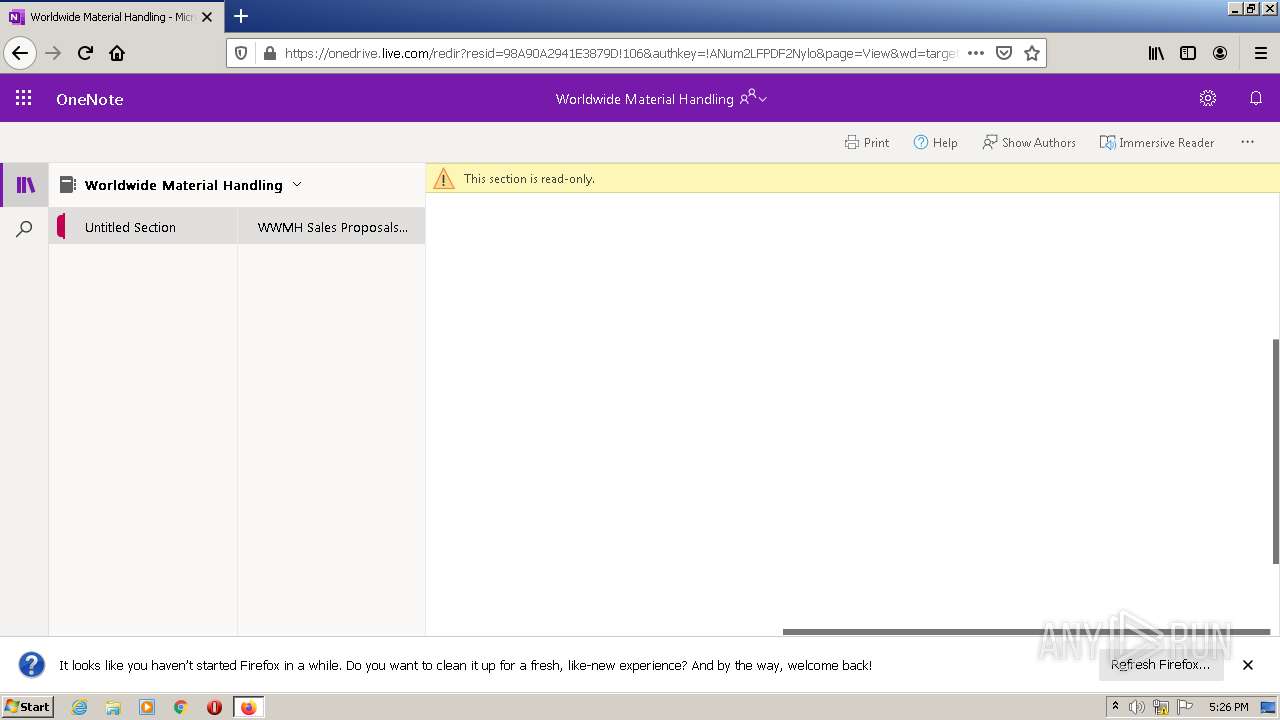The image depicts an open browser tab showcasing an interface reminiscent of older web browsers, such as early versions of Firefox or Internet Explorer. The browser window features the classic gray minimize, maximize, and close buttons, indicative of a dated design. In the upper left-hand corner, a tab displays a purple "N" and the title "Worldwide Material Handling."

The browser contains navigational buttons including back, forward, refresh, and home icons. The URL bar indicates "https://onedrive.live.com" with a redirect in place. Adjacent to the URL bar, there are icons for favorites, extensions, and profile options.

Directly below the URL bar, a purple-bordered header reads "OneNote - Worldwide Material Handling" with icons for a cogwheel (settings) and notification. The interface offers options such as Print, Help, Show Authors, and an Immersive Reader. Below this section, labeled "Worldwide Material Handling," is a hierarchy of sections including "Untitled Section" and "WWMH Sales Proposals."

The main content area of the page features a yellow caution icon and a message indicating that the section is "read-only." Accompanying this message is a prompt stating, "It looks like you haven't started Firefox in a while. Do you want to clean it up for a fresh, like-new experience?" Following this is a welcoming note, "Welcome back!" with a button labeled "Refresh Firefox" inviting the user to optimize their browser experience.